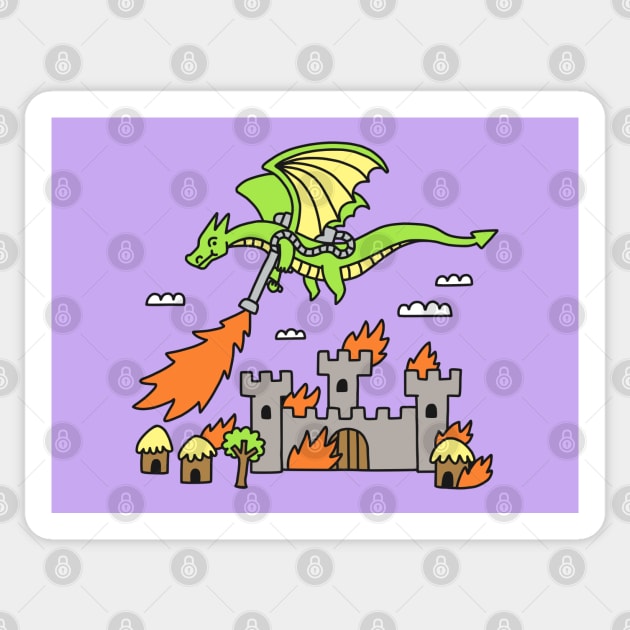A vibrant, digitally illustrated scene depicts a bright lime green dragon with four limbs, two wings, and two small horns soaring through a lilac purple sky. The dragon, positioned centrally towards the top, wields a gray flamethrower, its hose connected to a canister on the dragon's back, unleashing flames upon a gray stone castle and the surrounding area below. The medieval castle, with its three towers and a central round wooden door, is engulfed in fire. Nearby, three small huts with green, straw-like roofs and a single green tree with a brown trunk are also ablaze. The light gray background of the image is overlaid with a repetitive watermark featuring a small gray padlock within a gray diamond pattern. The entire scene is framed by a white border, enhancing the whimsical and chaotic intensity of the clipart-style artwork. A few white clouds linger in the sky, adding depth to the fantastical conflagration.